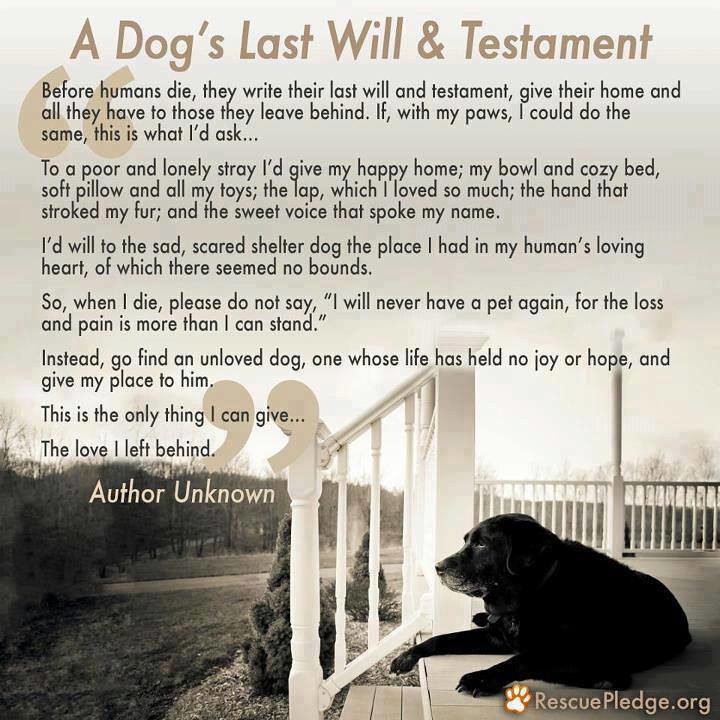The image is an inspirational poster predominantly with shades of white, darkish white, and earthy tones, transitioning three-quarters of the way down to a serene scene of grass and trees. In the bottom right corner, a black dog sits on a white porch with white fencing, gazing pensively into the distance. Overlaid in an orange font at the top of the poster are the words "A Dog's Last Will and Testament." Below, the text reads:

"Before humans die, they write their last will and testament, giving their home and all they have to those they leave behind. If with my paws I could do the same, this is what I'd ask: To a poor and lonely stray, I'd give my happy home, my bowl and cozy bed, soft pillow and all my toys, the lap which I love so much, the hand that stroked my fur, and the sweet voice that spoke my name. I'd will to the sad, scared shelter dog the place I had in my human’s loving heart, of which there seemed no bounds. So when I die, please do not say, 'I will never have a pet again, for the loss and pain is more than I can stand.' Instead, go find an unloved dog, one whose life has held no joy or hope, and give my place to him. It's the only thing I can give — the love I left behind." 

The author is unknown. At the bottom right, the website RescuePledge.org is noted, tying the heartfelt message to a cause for animal rescue.